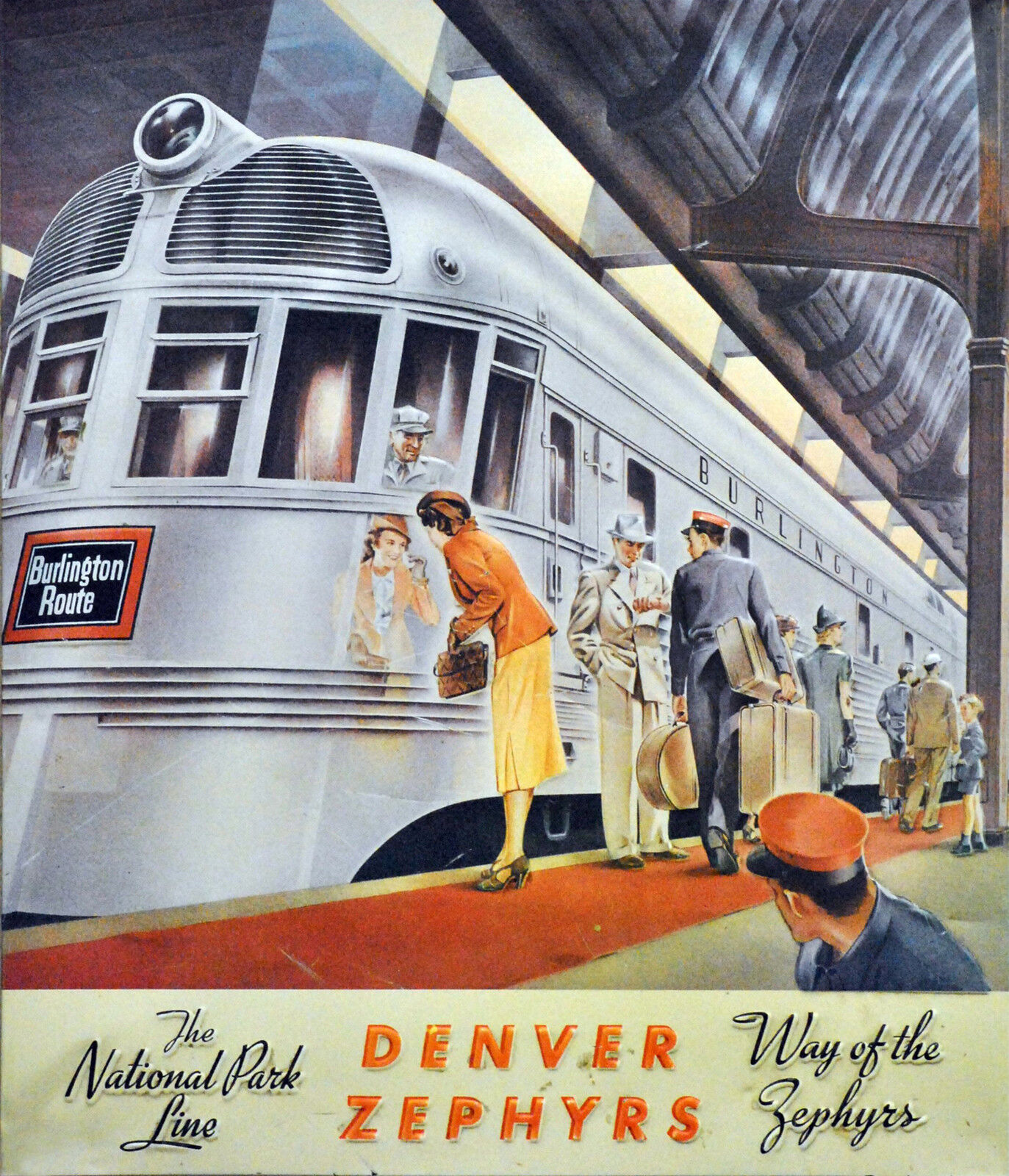This vintage advertisement, likely from the 1930s or 1940s, showcases the sleek, Art Deco style Denver Zephyrs, part of the National Park Line. The image, reminiscent of a National Geographic spread, features an imposing, rounded train adorned with a red and black "Burlington Route" sign at the front. The train station platform is topped with a corrugated steel archway and marked by a safety barrier red line along its edge. 

At the head of the train, we see two engineers, one prominently looking out from the window, dressed in a white jacket and conductor's cap. Reflecting in the train's shiny surface, a stylish woman in an orange jacket with a yellow knee-length skirt and black high heels attends to her makeup. She is carrying a handbag and stands with poise, oblivious to the bustling surroundings.

Nearby, a man dressed in a white suit and fedora checks his watch. Another porter, distinguishable by his red cap, hauls luggage towards the train. The background is animated with several other adults and a child, going about their activities. Another porter is in the foreground, seemingly resting while glancing back at the train. Throughout the scene, the dynamic layout and busy platform create a vivid snapshot of travel glamour from a bygone era.